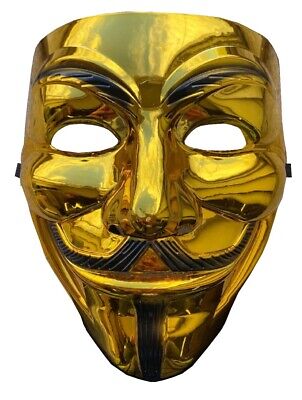This high-resolution, professionally taken image depicts a gold theater-style mask set against a clean, white background. The mask, reminiscent of the "V for Vendetta" style, features a bright, shiny gold color akin to 14 or 18 carat gold. It has two open eye sockets and small black hooks at the ear sections. The eyebrows are arched and black, while the face displays high cheekbones and a broad nose. A distinct three-lined black mustache extends from beneath the nose, arching over the mouth and reaching under the cheekbones, framed by a narrow black goatee line running from under the lips to the tip of the chin. The mask's jawline tapers into an upside-down triangular shape, and its smiling mouth exudes a dark, grimacing quality. The overall appearance is both striking and slightly eerie, capturing the essence of theatrical and enigmatic human expression.